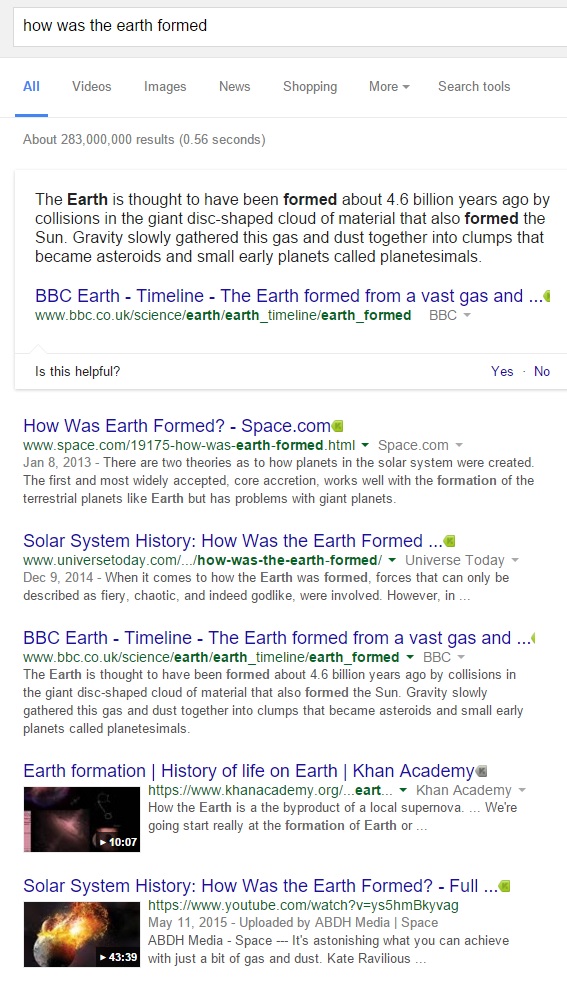A screenshot of a Google search query asking "how was the Earth formed" is displayed. The highlighted answer, derived from BBC Earth - Timeline, states that the Earth is believed to have formed approximately 4.6 billion years ago through collisions in a giant, disk-shaped cloud of material that also created the Sun. Gravity gradually pulled this gas and dust together into clumps that eventually became asteroids and small early planets, referred to as planetesimals.

Below the answer, the BBC Earth link is provided for further reading. The webpage interface shows iconic tabs for 'Videos,' 'Images,' 'News,' 'Shopping,' and a dropdown menu labeled 'More.' Additionally, there's a 'Search Tools' link. A bar below these options indicates that the search yielded about 283 billion results, achieved in 0.56 seconds.

Following the featured snippet, other related search results are listed, including links to articles from Space.com, Universe Today, and the BBC Earth link mentioned earlier. Two videos are also suggested: "Earth Formation: History of Life on Earth" from Khan Academy and "Solar System History: How is the Earth Formed?" available on YouTube.